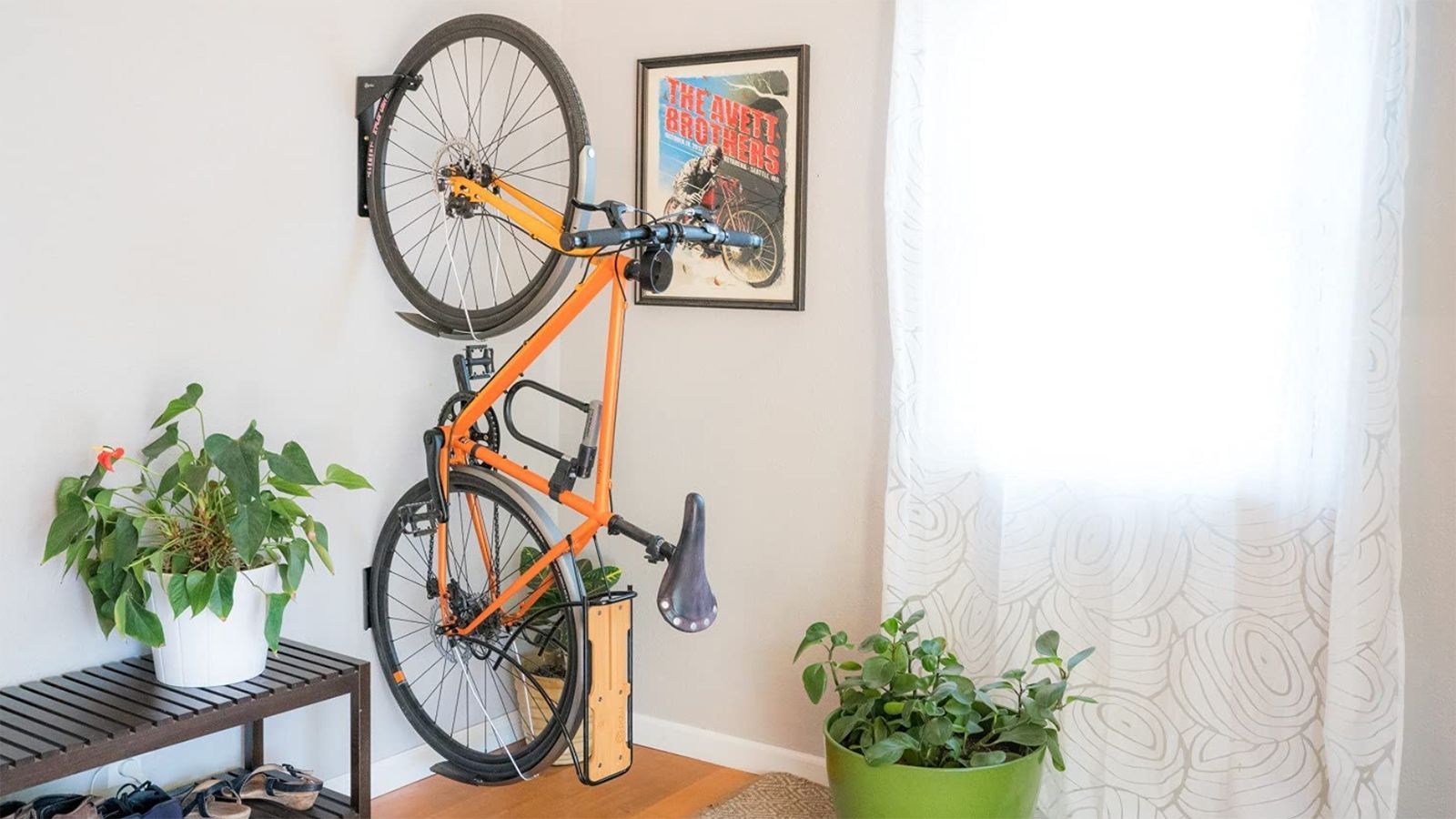The photograph captures a detailed scene of a home interior featuring a vibrant orange bicycle with black handlebars and wheels, mounted vertically on a light gray wall. The bike is secured by a two-section bike mount, with the front tire held by the upper part and the back tire resting on the lower section. Silver fenders and a black leather seat with bolts accentuate the bike. To the left of the bike, a wooden slatted shoe holder is pushed against the wall, topped with a potted plant in a white pot. Another potted plant in a green pot adds a touch of nature to the room. The light filters through a window behind a semi-transparent white curtain adorned with a gray pattern, illuminating a framed painting that references "The Omni Brothers." The overall ambiance combines elements of practical storage, art, and greenery in a cozy indoor space.